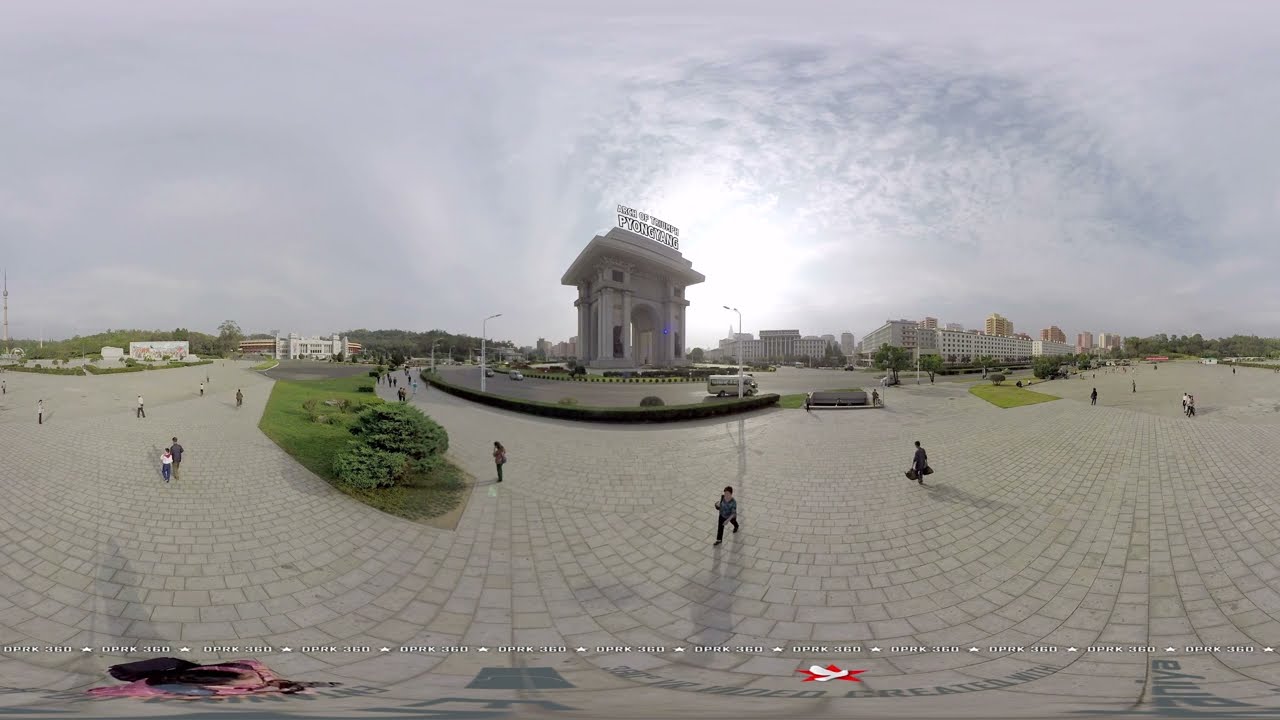The image captures a wide-angle view of a large, open plaza in an urban area on a cloudy day, with off-white and gray tile covering the ground in a circular pattern. Various people are walking around the plaza, which is punctuated by sections of greenery, including small shrub-like trees. Dominating the center of the image is a grand, white structure that resembles the Arc de Triomphe, potentially made of marble. This tall arch features two windows at the top, flanked by large door-like openings at the base on either side of the arch. The word "Pyongyang" is prominently displayed atop the structure, indicating the location. A roundabout seems to encircle the structure, suggesting areas where cars can pass through. The city skyline with several buildings is visible in the background under a cloudy, grayish sky with the sun faintly shining through. The overall scene depicts a bustling city square in Pyongyang, North Korea, with low vehicular traffic and a blend of urban elements and natural spots.